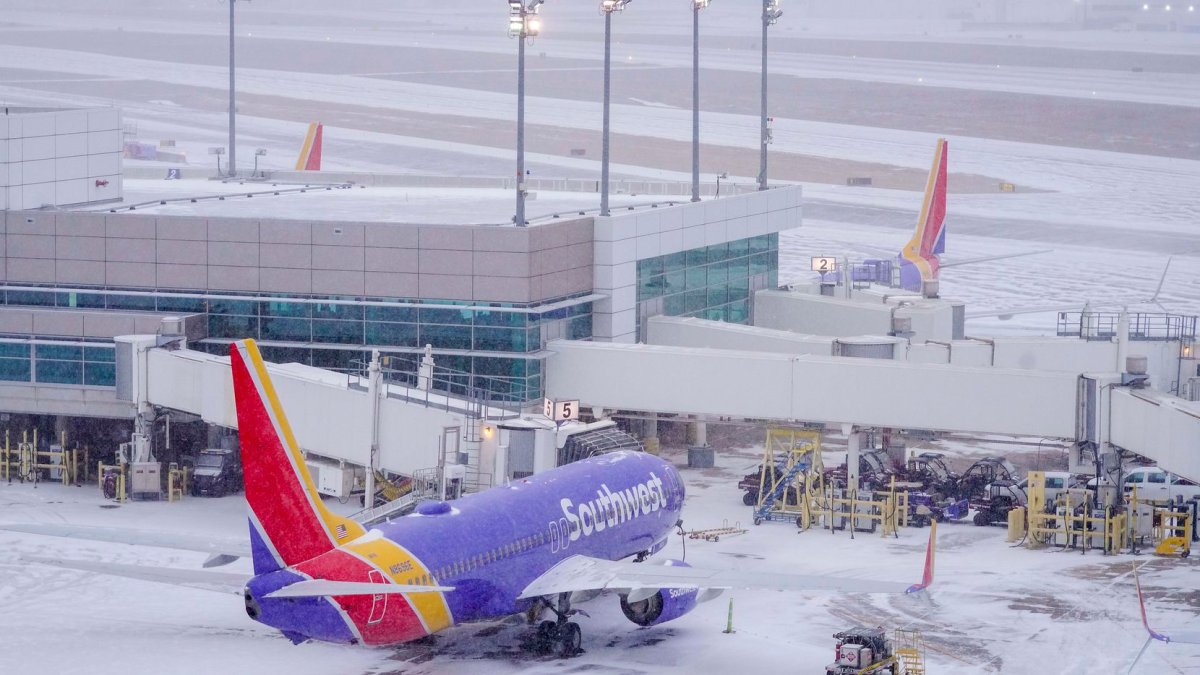This is a detailed color photograph of an airport terminal in winter, taken from an elevated, possibly aerial, viewpoint. The image captures a snowy landscape with a terminal building prominently featured in the center. The terminal building has blue-tinted windows covering much of its structure, white cinder blocks, and is topped with multiple tall poles with lights. Below the windows, there is a garage level housing various service vehicles and yellow safety barricades.

In the foreground, a Southwest Airlines plane, characterized by its blue body, white wings, and engines, is docked at the gate. The jetway extends from the building to the aircraft, which displays "Southwest" in white text across the fuselage. The plane’s tail proudly sports red and yellow stripes that run down across the body. Its black wheels are visible on the snow-covered tarmac.

The backdrop reveals the tail fins of two other Southwest planes with matching livery, one partially obscured by the terminal while the other peeks out from behind the building's right edge. The surrounding runways and taxi areas are blanketed in snow, emphasizing the cold, wintry conditions. The sky above appears hazy and cloudy, adding to the stark winter atmosphere.